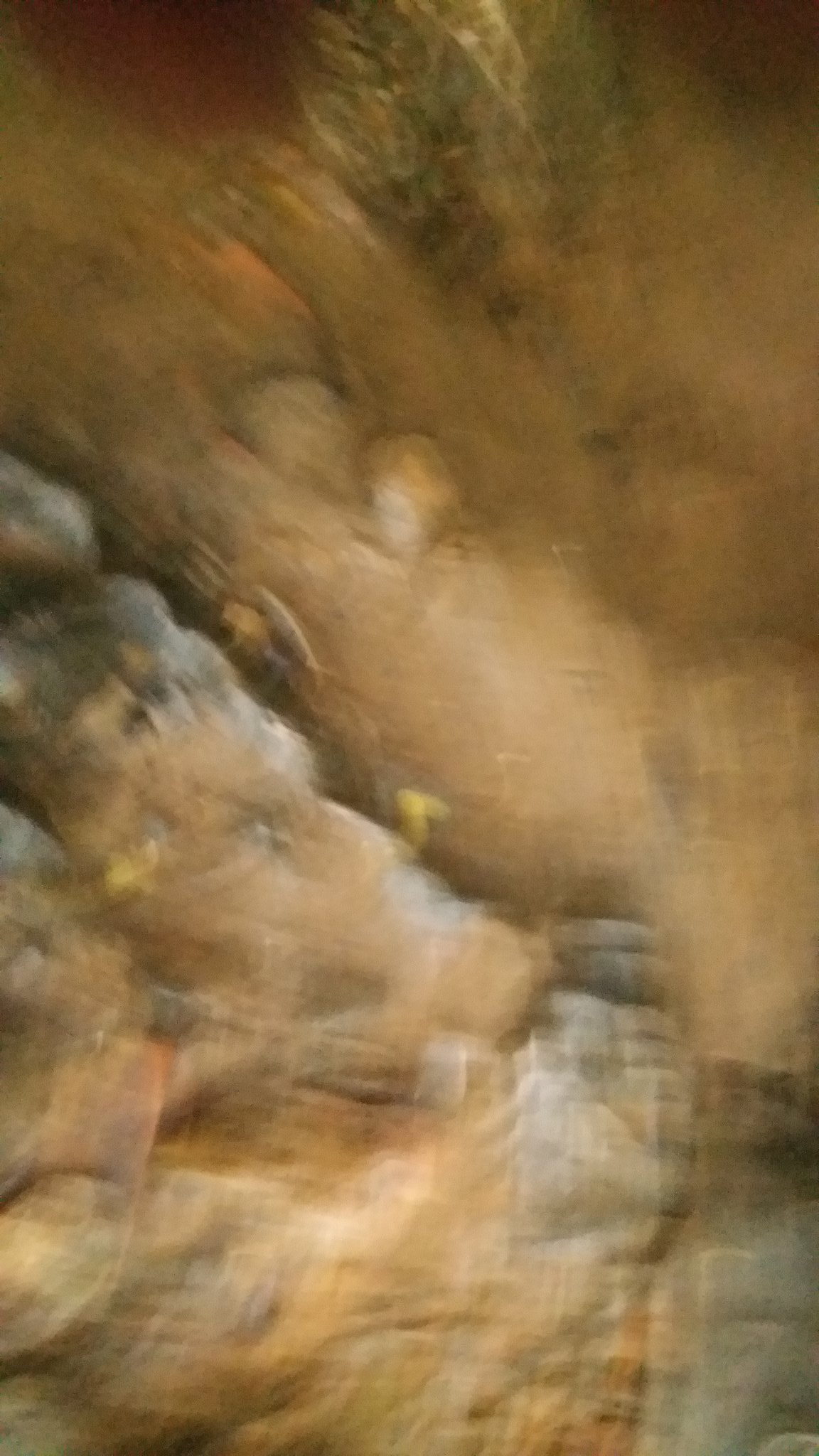The image depicts an extremely blurry and out-of-focus scene characterized by a series of indistinct brown and gray shapes. The top of the image features a very dark area and what appears to be a tuft of grass or a bush. Below it, there is possibly a rock. The bottom section of the image is lighter in contrast, incorporating a mix of tan and gray colors that resemble smoke. On the bottom left, there's a small brown square shape, while the bottom right contains a somewhat pointy shape. The lower half of the image showcases a lot of bubbly-shaped objects, primarily in gray towards the right and with an orange tint on the left. There is also a faint white line separating some of the colors in the image. The upper corners are dark brown, adding to the overall indistinct and ambiguous nature of the scene.